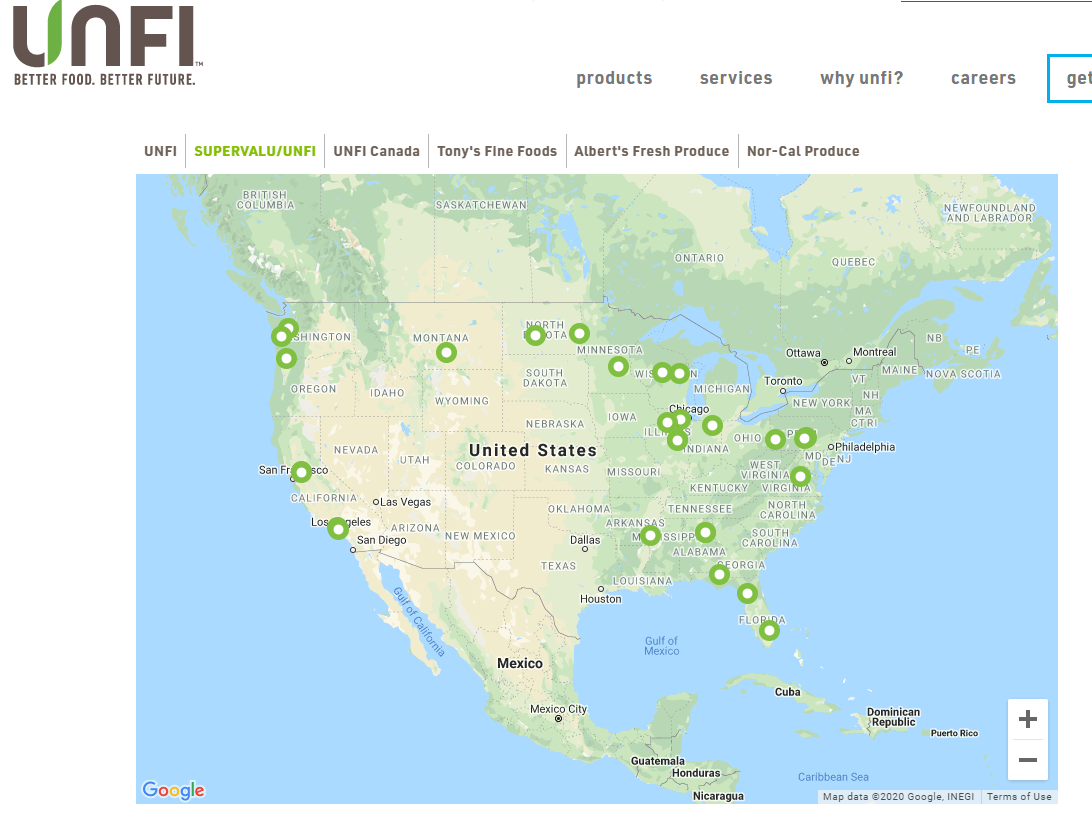The image depicts a web page serving as a locator tool for UNFI, a company that promotes "Better Food, Better Future." The background of the page is white, with the company's logo and slogan prominently displayed in bold black lettering at the top left. Adjacent to the logo, several navigation options are listed in smaller black text: Products, Services, Why UNFI?, Careers, and a partially visible button labeled "GET" highlighted with a blue line, suggesting it is part of a blue box.

Below this navigation bar is a second line of tabs that segment UNFI's services, including Super Value UNFI in green lettering, UNFI Canada, Tony's Fine Foods, Albert's Fresh Produce, and NorCal Produce. The central feature of the page is a large map that spans North America, focusing on Canada, the United States, and Mexico. The map is marked with numerous green dots, indicating the locations of UNFI's various operations, which appear to be concentrated primarily within the United States. No locations are highlighted outside of the U.S. within North America as indicated by the absence of green dots in Canada and Mexico.